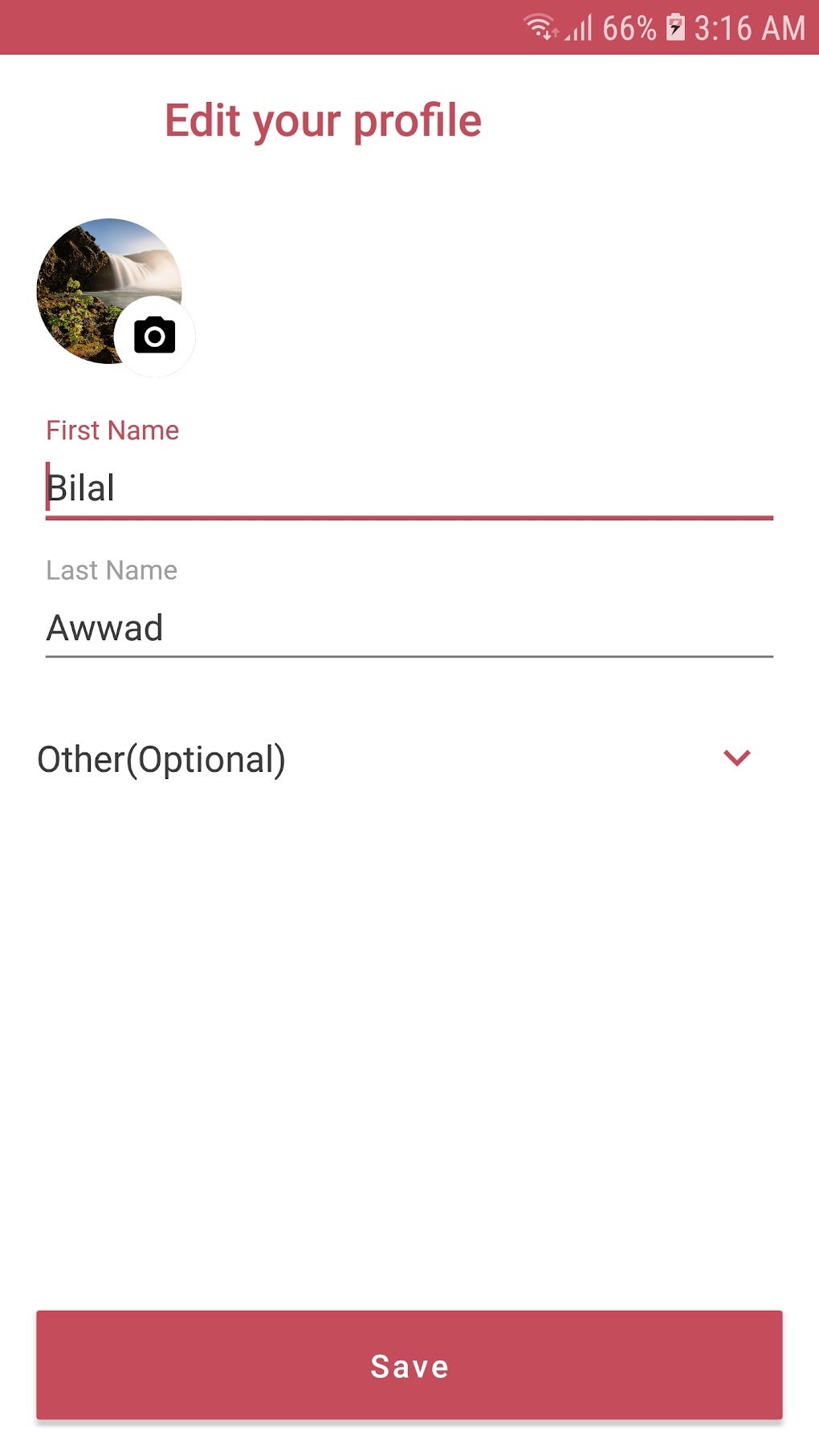The image displays a detailed user interface screen with various elements. At the top left corner, a red bar is visible, indicating a 3 out of 4 status, possibly related to battery or signal strength. Adjacent to it is a full Wi-Fi signal icon. The banner displays the time as 6:00 AM, accompanied by a notice at 6:03 AM stating "I need your profile." 

Below these elements, there is a scenic background featuring a serene lake with a waterfall, under a clear blue sky, giving a calm and natural feel. Within the interface, there is a text field with a placeholder labeled "First Name," followed by another field labeled "Last Name" containing the text "Awad." A gray line separates these fields.

Additionally, there is an optional text field titled "Other," which is accompanied by a parenthetical note indicating its optional nature. To the right of this field, there is a red drop-down menu. Below these fields, there are buttons labeled "View," "Save," and "Send," which are colored with green, blue, and red squares respectively. These buttons suggest options for saving the profile details or sending the information.

At the top left corner of the screen, there is an avatar icon, which likely allows the user to click and upload or change their profile picture via an embedded camera option. The overall layout suggests a user-friendly interface designed to edit and update a user's profile information seamlessly.